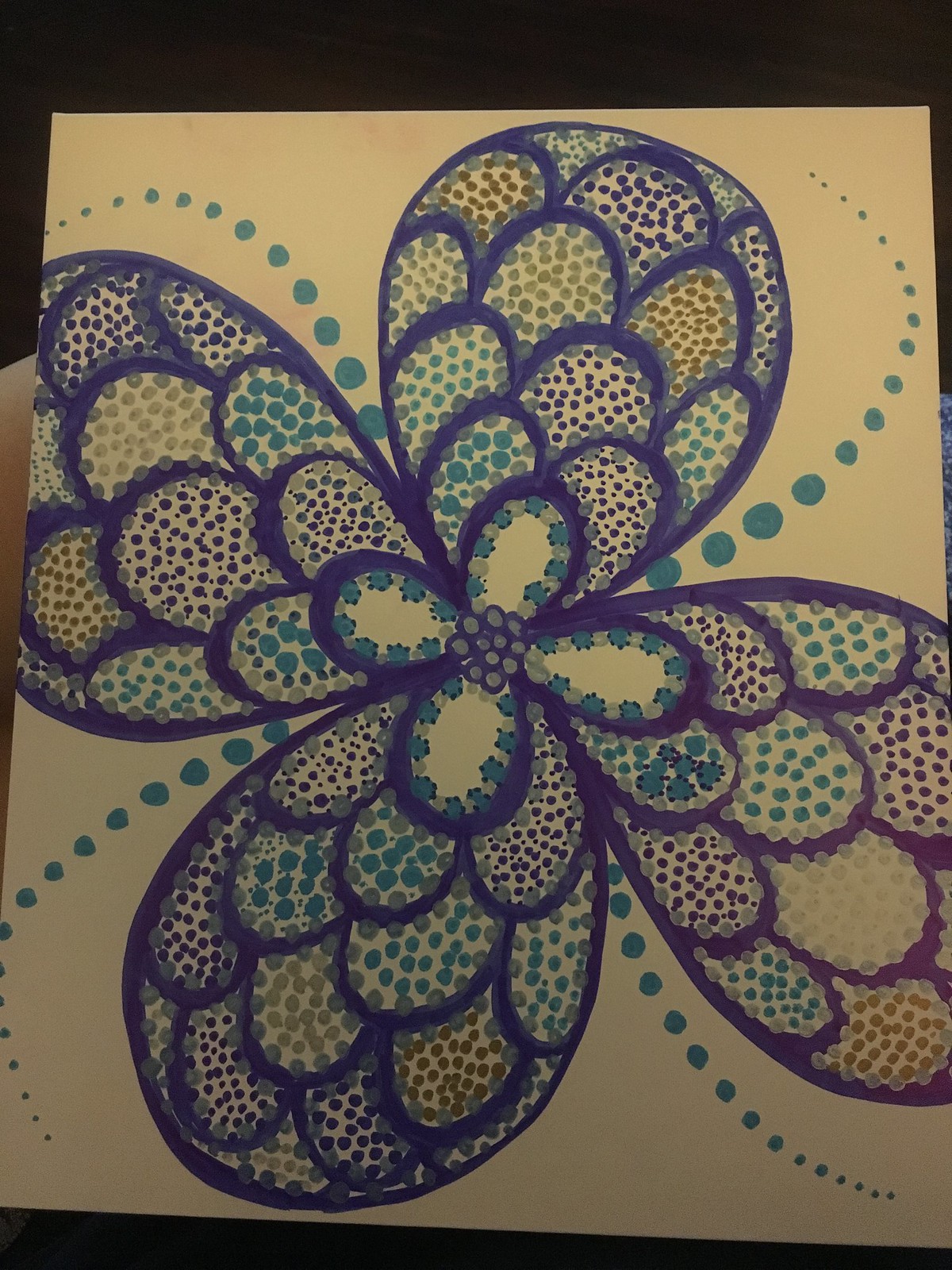This image depicts a detailed watercolor drawing on a piece of white poster board, which resembles a large, colorful flower or butterfly with four wings or petals. Each petal radiates from a central area that looks like a cluster of grapes in violet, outlined with dark purple. Surrounding this central cluster are four inner petals lined with dark blue and violet dots edged in dark purple. Beyond these are four larger petals, each featuring egg-like shapes filled with dots in various colors such as purple, yellow, cyan, gold, dark brown, and gray, each accented with purple. The colors throughout the drawing include shades of purple, aqua blue, yellow, green, teal, light brown, and gray. Aqua-colored dots are a prominent feature, forming patterns that start larger near the center and trail off smaller as they extend to the edges of the petals. This intricate and colorful design creates a vibrant visual experience, blending floral and butterfly-like elements.